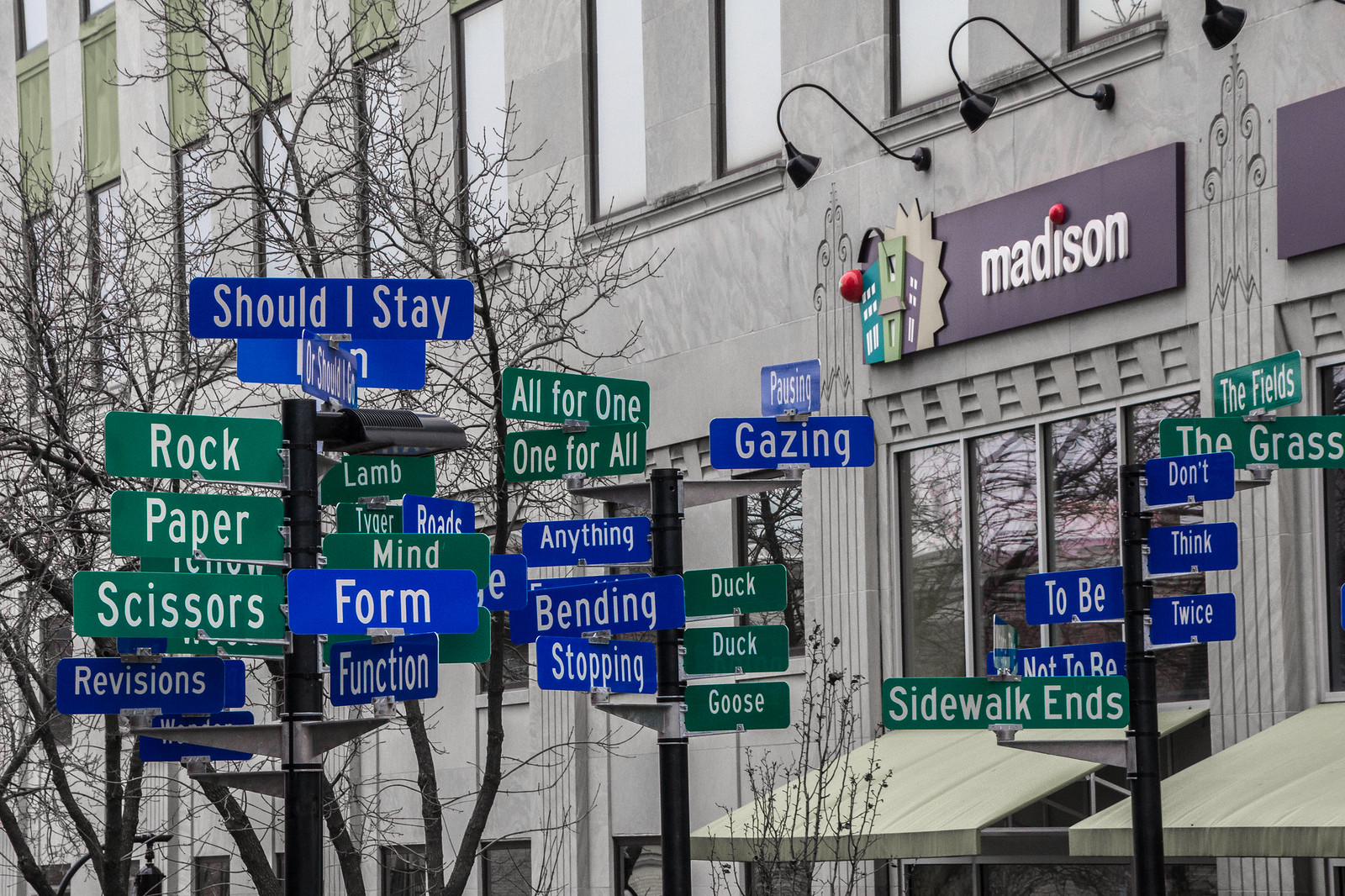The photograph features an outdoor scene captured in front of a large, greenish-gray building identified by a black and white "Madison" logo with a dot over the "i." The building showcases multiple windows and a canopy. Centered in the image are numerous blue and green street signs mounted on metal poles, lending a surreal and cluttered effect to the scene. These signs bear a variety of whimsical and non-traditional traffic instructions such as "rock," "paper," "scissors," "should I stay," "form," "function," "bending," "stopping," "duck, duck, goose," "sidewalk ends," and more. The setting conveys a mix of curiosity and absurdity, enhanced by the unorthodox and playful messages on the signs against the backdrop of the commercial building.